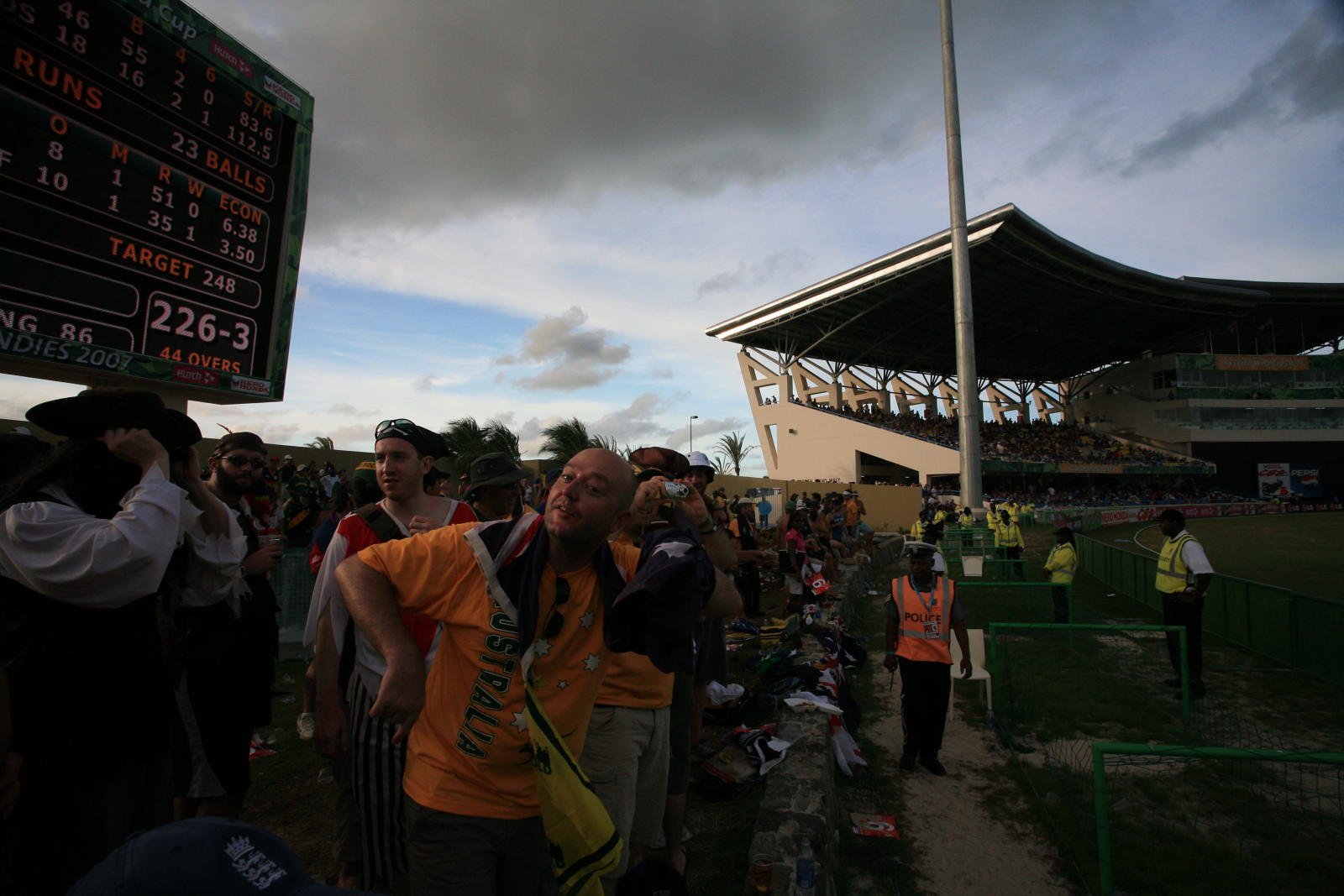This photograph captures an outdoor evening event at a large stadium, possibly a cricket game given the scoreboard's unique metrics like "23 balls," "226 over," and "target 248." The scene features a two-tiered seating structure with a hard tent-like canopy overhead. The sky is a mix of dark gray clouds and patches of blue in the distance, suggesting an impending rain. 

On the right lies a flat, green circular field bordered by a green metal fence. Numerous security personnel in yellow vests are lined up along this fence, with one individual in the middle wearing an orange vest emblazoned with the word “Police.” The left side of the image is packed with disheveled fans in colorful attire, some standing, others sitting, against a backdrop of noticeable debris and trash. A bald man in an orange t-shirt poses for the camera amidst the audience. 

A black scoreboard is situated in the upper left corner, further emphasizing details unique to a cricket game. The overall atmosphere portrays a lively, albeit slightly chaotic, sporting event under a dramatic evening sky.